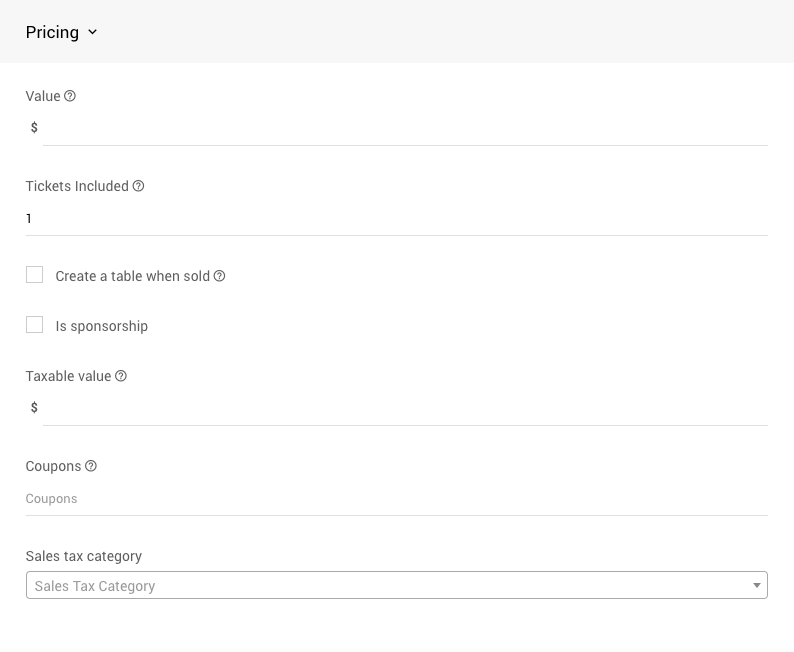The image features a form on a white background, detailing various aspects related to pricing. A gray header at the top prominently displays the word "Pricing" in bold black text, accompanied by a downward-pointing arrow.

Below the header, the form is structured into several fields:

1. **Value**: Denoted by a question mark next to a dollar sign, suggesting a placeholder for the value. This field is currently empty.
2. **Tickets Included**: Marked with a question mark, this field includes an input box where someone has entered "1".
3. **Create a Table When Sold**: This field poses a question and includes a checkbox, which remains unchecked.
4. **Sponsorship**: Another checkbox field that remains unchecked, indicating no sponsorship is selected.
5. **Taxable Value**: Labeled with a question mark and an empty input box for a dollar amount.
6. **Coupons**: This section is indicated with a question mark and a circle, suggesting the potential inclusion of coupons, but no coupons have been added.
7. **Sales Tax Category**: This field offers a drop-down menu for selecting a tax category, but it is currently set to the placeholder text "Sales Tax Category", with no selection made.

Overall, the form appears mostly unfilled, indicating that the majority of the fields require input or selection.